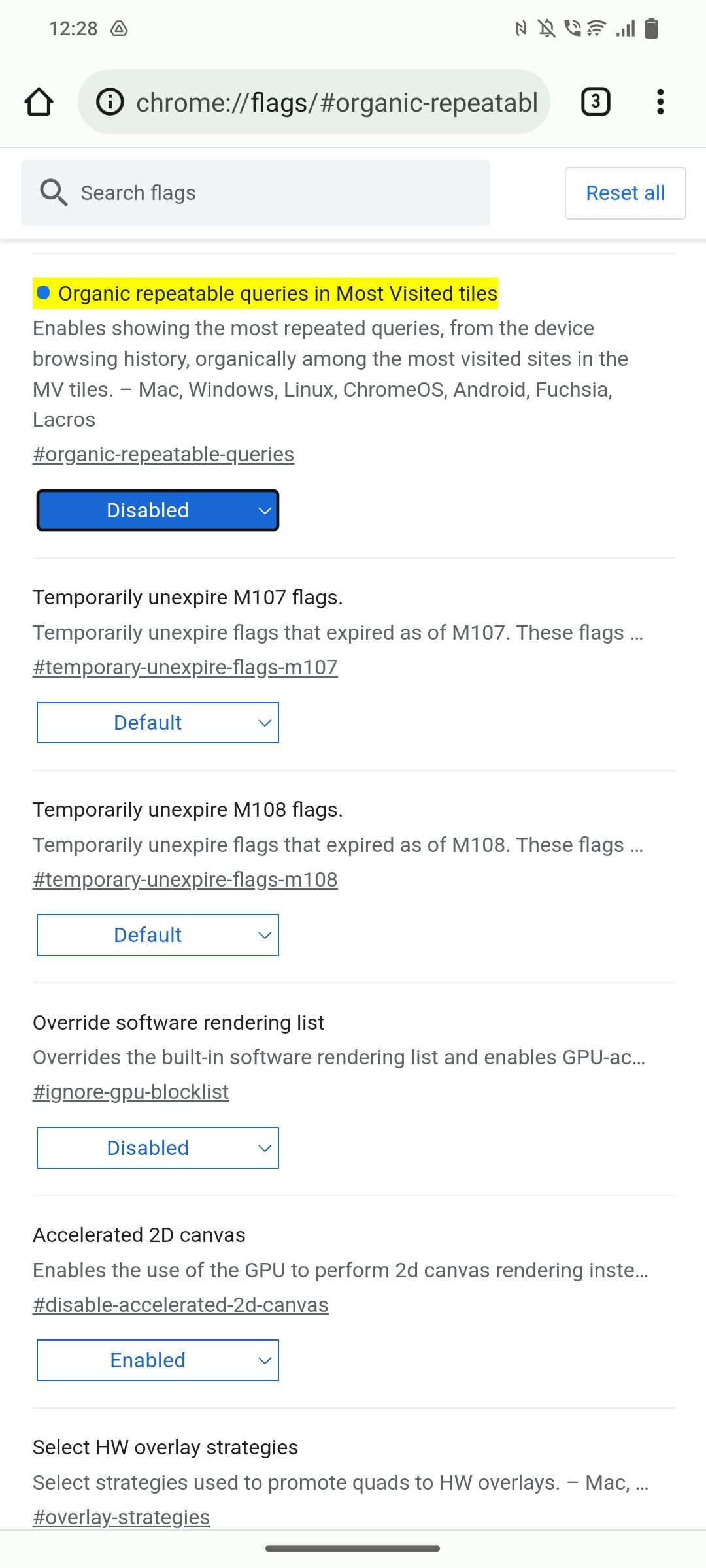A detailed descriptive caption for the provided image would be:

"Screenshot of search results in a mobile application displayed on a white background. At the top, a header with a greenish background features mobile phone icons and a medium gray house icon on the left. Adjacent to the house icon is a greenish dark gray URL bar with rounded edges, marked on the left by a black eye icon enclosed in a circle. The URL bar contains gray text that reads 'chrome://flags/#organic-repeatable', although some text is cut off. To the right of the URL bar, a black square with rounded corners displays a '3' in the middle, followed by a vertical stack of three black dots.

Below this header, the main part of the page starts with a light gray search bar on the top left, featuring a medium gray magnifying glass icon and the text 'Search flags' in medium gray. Adjacent to the search bar, a white button with a thin light gray outline bears the blue text 'Reset all.' A medium-width light gray line separates this section from the content below, followed by a very thin light gray line that doesn't traverse the full width of the page.

The search results are organized below these lines, each separated by thin light gray lines. The first search result, highlighted in yellow, shows black text with a blue dot to the left, stating 'Organic repeatable queries in most visited tiles.' Below this, in light gray text, is the description: 'Enables showing the most repeated queries from the device's browsing history organically among the most visited sites in the MV tiles - Mac, Windows, Linux, Chrome OS, Android, Fuchsia, Lacrosse.' Further below, the text 'chrome://flags/#organic-repeatable-queries' is underlined. A blue button with white text labeled 'Disabled' is located beneath this text, accompanied by a downward-pointing white arrow surrounded by a black outline. Similar search results follow below."